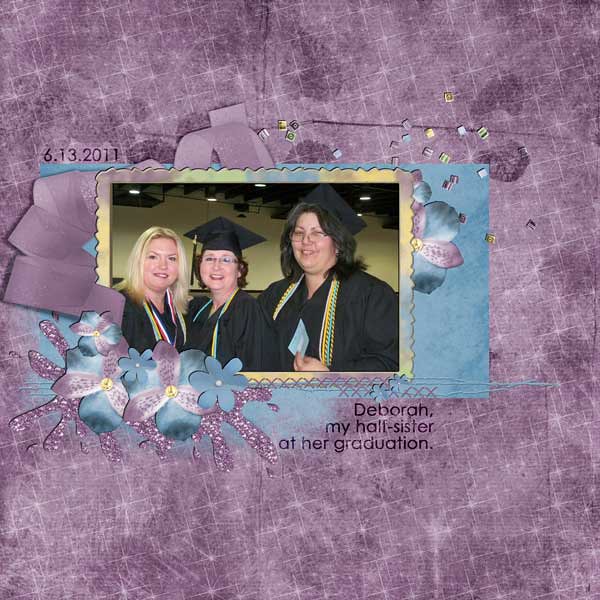This image features a scrapbook page with a vibrant purple and blue background, decorated with glittery, white markings and purple and blue flowers. At the center, slightly left and above the exact midpoint, is a colorful framed photograph of three women at a graduation. The frame itself is light blue with floral decorations in the bottom left and upper right corners. 

In the photograph, the woman on the left has shoulder-length blonde hair and wears medals or ribbons around her neck, paired with a black robe. She is slightly turned to the right but looks forward, smiling. The central figure, clearly the graduate, dons a black cap with a tassel on the right, glasses, and a black robe with a yellow ribbon or tassel around her neck. She has short brown hair and is also smiling, facing forward but slightly turned to the left. The tallest woman stands on the right, also smiling. She has shoulder-length black hair, wears glasses, and is dressed in a black robe with a graduation cap. She has a yellow ribbon or tassel around her neck and holds a small card in her left hand.

The background of the photograph shows a yellow wall with ceiling lights. The date '6-13-2011' is written in black ink at the top left of the photograph, and beneath it, in black letters, it reads: 'Deborah, my half-sister, at her graduation.' The dominant colors in the image and the scrapbook page are blue, purple, white, black, and yellow.